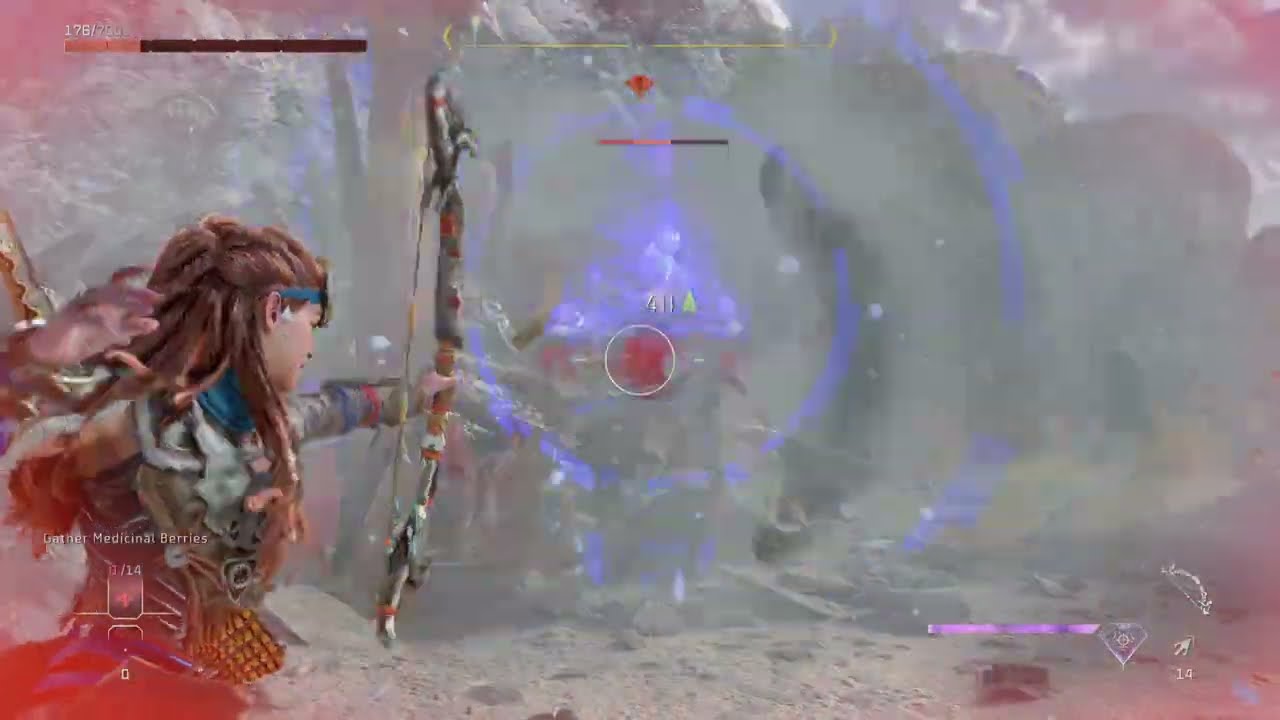The screenshot captures an action-packed scene from a video game featuring a female character with long hair pulled back into ringlets, adorned with a blue headband. Positioned on the far left side of the screen, she is depicted in a dynamic stance, having just released an arrow from her bow, held in her left hand with her right hand drawn back near her ear. Her colorful armor, featuring hues of browns, grays, bluish-green, and splashes of pink and red, hints at a protective chest plate and a blue and red strap around her wrist. The background showcases a mix of grays, purples, and greens, adding to the sense of a historical yet slightly futuristic setting. Central to the image is a target indicator, marked by a red blotchy circle surrounded by purple rings, signifying where the arrow was aimed. A life meter above her shows the number 176, indicating she has less than half her health remaining, while text at the bottom mentions "medicinal berries" with a count of 0/14. The combination of vivid colors and dynamic composition underscores the intense action of the scene.